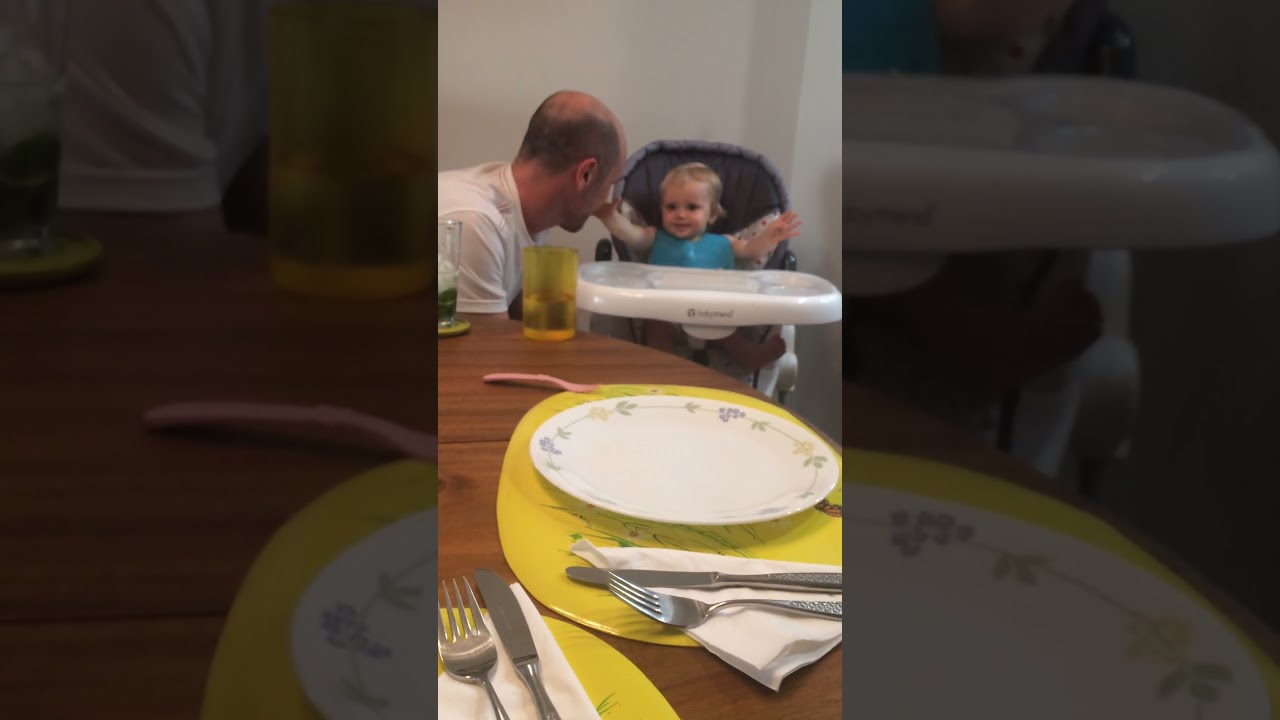In a triptych of images, the central photograph depicts a tender moment between a father and his young daughter at a dining room table. The man, dressed in a white t-shirt and partially bald, sits on the left side of the frame, attentively engaging with his smiling toddler. She, with her arms joyfully stretched upward, sits in a black high chair with a white tray, donned in a blue shirt, her light blonde hair aglow. The table before them is a warm wood tone, set with yellow placemats, and features formal place settings, including plates, silverware, and napkins. A round table in the foreground also showcases detailed settings, including two plates with knives and forks laid on white folded napkins. To the right of the scene, a yellow glass subtly adds to the composition. The background is defined by a simple white wall, focusing attention on the intimate interaction. Flanking the central image, the left and right panels are blown-up, darker, and overexposed sections of the original photograph, adding an abstract contrast to the detailed realism of the core image.